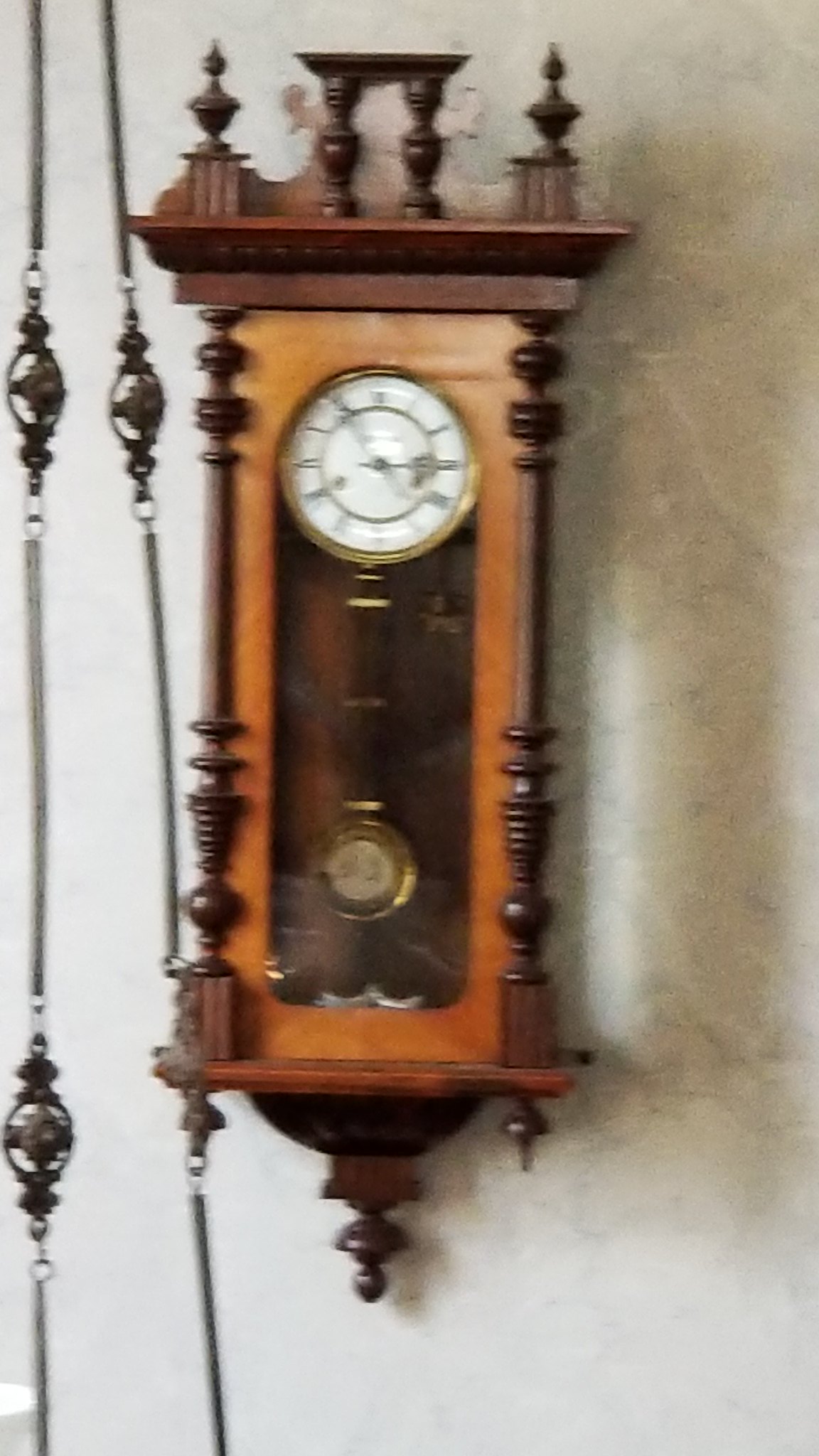An out-of-focus photograph features an antique clock mounted on a white, textured wall. The clock is crafted from wood and exhibits a two-tone design. Its front frame is a lighter shade of brown, while the top, columns, and base are a richer, darker brown, adorned with numerous spindles that enhance its classical aesthetic. The clock face is white and is marked with Roman numerals. Hanging below the clock is a pendulum that combines wooden elements with a gold face, which bears white lettering.